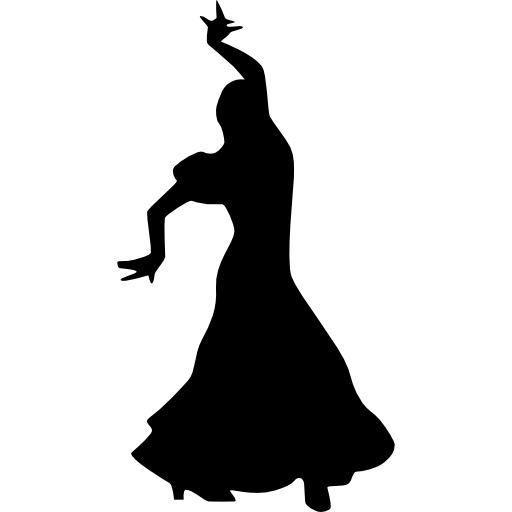The image features a simple yet striking black and white graphic design of a dancer's silhouette against a plain white background. The figure, likely female, is depicted in an elegant pose with her left hand raised above her head, extending her index and pinky fingers upward while bending the other fingers perpendicular to the right. Her right arm is gracefully extended behind her, with the fingers slightly splayed. The dancer appears to be wearing a long dress that flows past her ankles and high-heeled shoes, emphasizing the poised nature of the silhouette. The abstract design leaves the interior of the black silhouette entirely devoid of details, focusing solely on the expressive form and dynamic posture of the dancer.